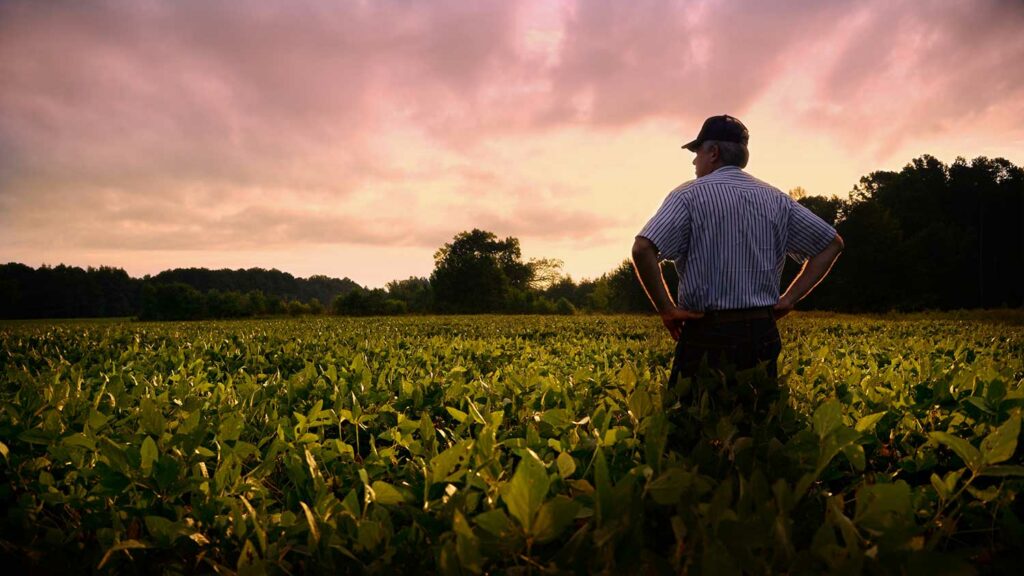In this horizontally aligned rectangular picture, an older man, likely in his 50s, stands in contemplative observation of his expansive field, possibly soybeans. He is wearing a black baseball cap, a blue and white vertically striped short-sleeve button-down shirt, and black pants. With his hands on his hips, he gazes over the dense green vegetation that reaches up to his mid-thigh. The sky behind him is strikingly beautiful, suggesting either early morning or sunset, with a blend of yellow, pink, and purple hues amidst gray and brown clouds. In the far background, a line of tall trees spans across the image from left to right, with a notable height difference favoring the right side. Despite some insect-damaged leaves, the field of crops stretches out extensively, encapsulating the man's dedicated and reflective stance.